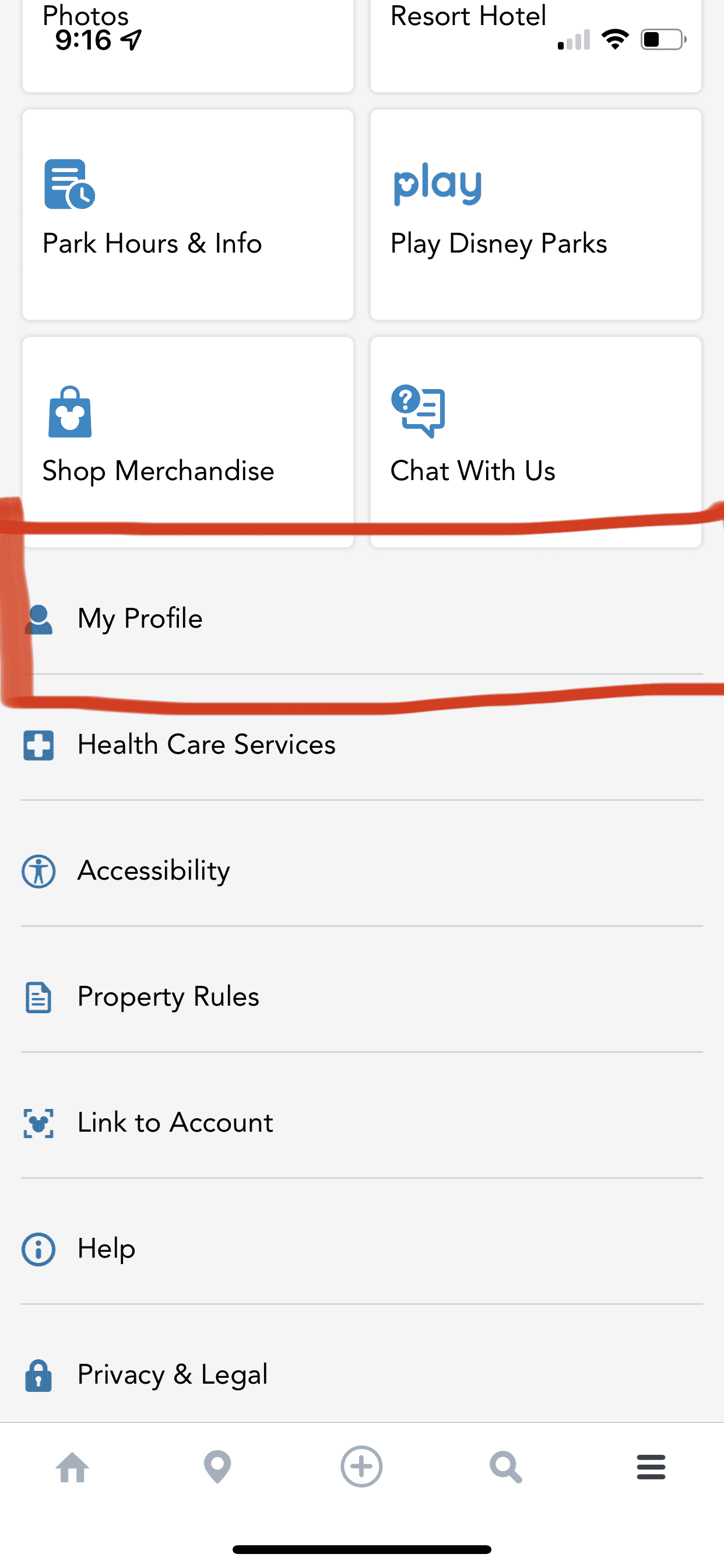The image depicts a screenshot from a Disneyland or Disney World mobile application. At the top left, the time reads "9:16 AM," accompanied by a location service icon. On the right side of the screen, connectivity indicators are visible, showing a signal strength icon with only one bar filled, a fully filled Wi-Fi icon, and a horizontal battery icon indicating 30% charge.

Below the status bar are six primary buttons displayed on a white background with black text:
1. Partially visible buttons: "Photos" on the left and "Resort Hotel" on the right.
2. Fully visible buttons:
   - A button featuring a blue document icon with a clock symbol at the bottom right, labeled "Park Hours and Info."
   - A "Play Disney Parks" button where the "P" incorporates a Mickey Mouse head, with the text in blue.
3. Another row of buttons includes:
   - A shopping button with a blue bag icon and a white Mickey head, labeled "Shop Merchandise."
   - A chat support button with a blue chat bubble featuring a white question mark, labeled "Chat with Us."

Below these buttons, a settings section includes labels with gray background separators:
1. "My Profile" with a profile icon, encircled messily in red marker-like ink.
2. "Health Care Services" with a blue square and white cross icon.
3. "Accessibility" with a blue circle icon showing a stick figure with outstretched arms.
4. "Property Rules" with a document icon featuring a folded corner.
5. "Link to Account" with a Mickey head icon.
6. "Help" with a blue circle icon housing an "i."
7. "Privacy and Legal" with a blue lock icon containing a white keyhole.

At the bottom of the screen lies a navigation menu on a white background with gray icons:
1. A Home icon.
2. A Location Services icon.
3. A circle with a plus sign.
4. A magnifying glass icon.
5. Three horizontal lines icon representing a dropdown menu.